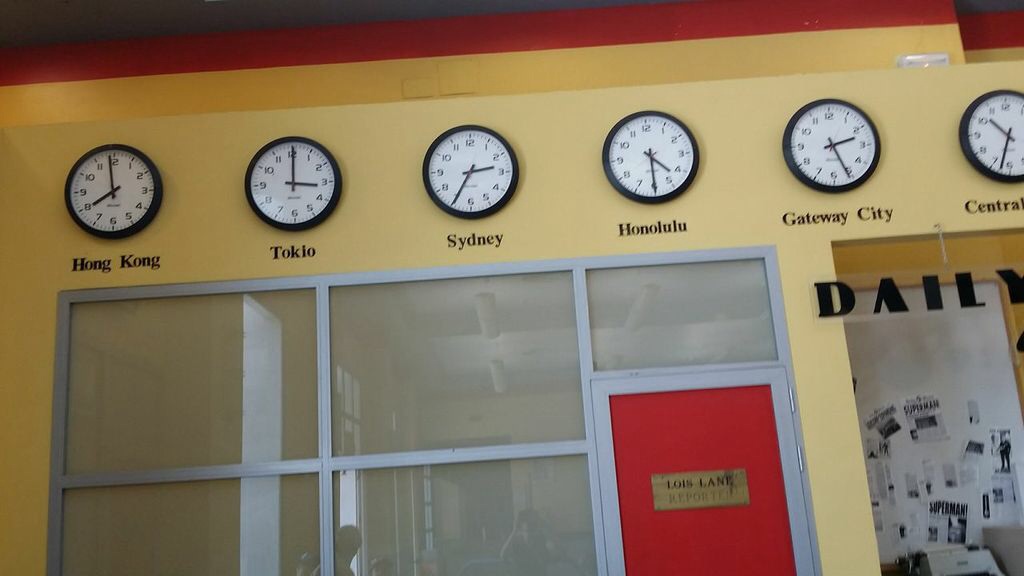In the image, we see a professional office setting featuring a prominent red door labeled "Lois Lane Reporter." The door is flanked by windows, which appear to be covered, likely for privacy or light control. Above the door, there is a row of six classic white clocks, each framed with a black circular casing. Each clock displays a different time, marked by standard numerals and equipped with minute and hour hands. The locations indicated by the clocks are Hong Kong, Tokyo, Sydney, Honolulu, Gateway City, and Central. The overall scene captures the essence of a busy, international news office, with Lois Lane's door suggesting a dedicated and perhaps high-profile journalist workspace. The details, such as the varied times on the clocks and the obscured windows, hint at the dynamic and fast-paced environment typical of a newsroom.